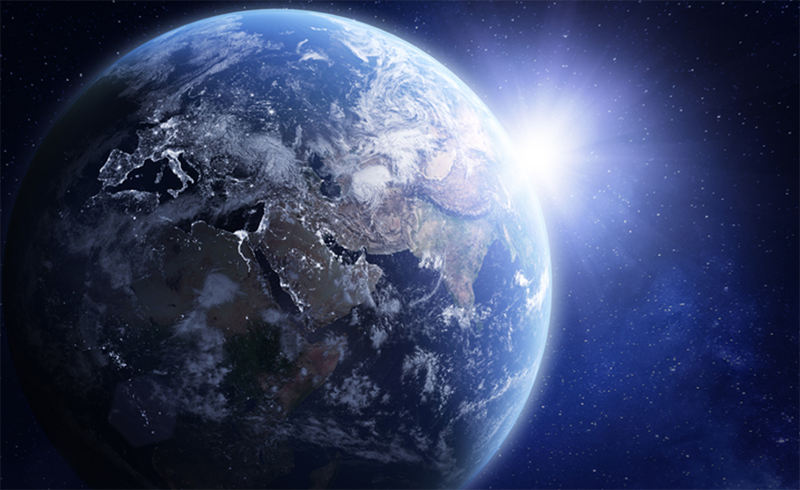This stunning photograph, captured from space either by a spacecraft or satellite, showcases Earth in all its splendor. The image prominently features the blue oceans and brown and white landmasses of the continents. In the upper left portion, the distinctive boot shape of Italy is visible, as well as Europe, which is outlined in white lights indicative of nighttime. The illuminated Suez Canal is also noticeable, adding to the intricate network of lights. An array of storms and cloud formations swirl above the Earth, adding dynamic elements to the scene. The planet is set against a deep midnight blue sky, dotted with tiny pinpoints of distant stars. On the right-hand side, the sun is seen rising, casting a brilliant white light with radiant beams extending outward, illuminating the edge of the Earth.